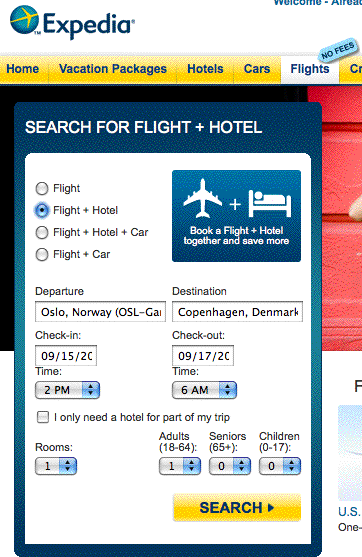An Expedia webpage is displayed prominently on the screen. In the top left corner, the Expedia logo is visible, featuring the word "Expedia" in dark blue and a circular icon with a yellow airplane inside. Directly below the logo are several navigation tabs, each with a yellow background and dark blue text. The tabs, from left to right, are labeled "Home," "Vacation Packages," "Hotel," "Cars," and "Flight," with the "Flight" tab highlighted in white.

A tag stating "No Fees" is positioned below the tabs. Beneath this, there's a search bar labeled "Search for Flight + Hotel," with selectable options for "Flight," "Flight + Hotel," "Flight + Hotel + Car," and "Flight + Car." The "Flight + Hotel" option is currently selected. To the right of the search bar, a blue square contains white icons of an airplane and a bed, accompanied by the text "Book a flight + hotel together and save more."

Further down, the departure and destination information are filled in as follows: the departure location is Oslo, Norway (OSL), with a check-in date of 19th July at 2 PM, while the destination is Copenhagen, Denmark, with a check-out date of 21st July at 6 AM. Below this, a checkbox option reads "I only need a hotel for part of my trip."

The form also includes details about room and passenger preferences: one room, one adult, zero seniors, and zero children. At the bottom right corner of the form, a prominent yellow button marked "Search" is ready to be clicked.